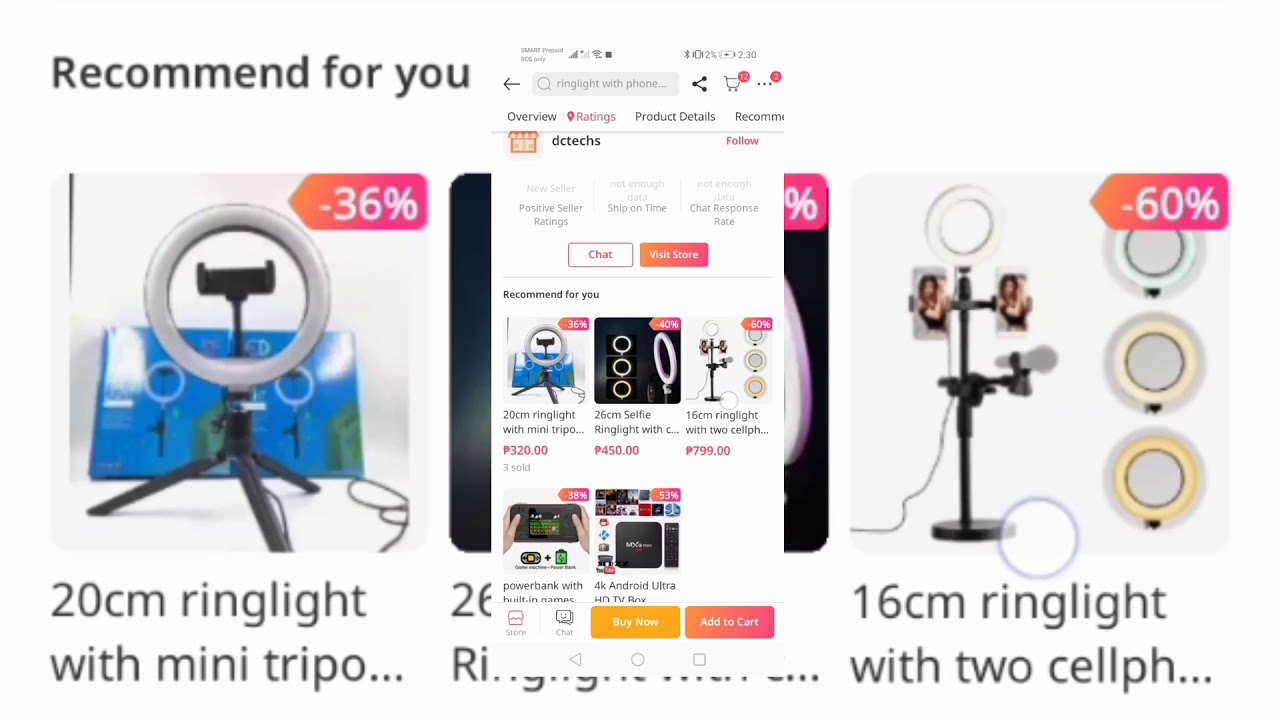Screenshot of a shopping website interface in landscape mode with an off-gray background. In the upper left-hand corner, "Recommended for You" is displayed, partially covered by a white pop-up menu. This pop-up menu features sections including Overview, Ratings, Product Details, and a search bar at the top. Below these sections, the menu continues in a single long column detailing various products.

Beneath the main menu header, there's a navigation option labeled "DC Techs" with additional options to chat or visit the store. Several recommended products are displayed below. On the bottom left-hand corner, there are two buttons: an orange "Buy Now" button and a gradient orange-to-red "Add to Cart" button.

The recommended products are shown on the left side, starting with a "20 cm Ring Light with Mini Tripod" advertised at a 36% discount, with its image displayed above. The next product in the list shows a 26% discount, but the image above it is unclear. The third item is a "16 cm Ring Light with Two Cell Phone Holders," available at a 60% discount, and the image indicates it also has a microphone holder. 

This setup suggests the interface might be part of a shopping app or extension, potentially Rakuten, that helps users find discounted products while they shop.